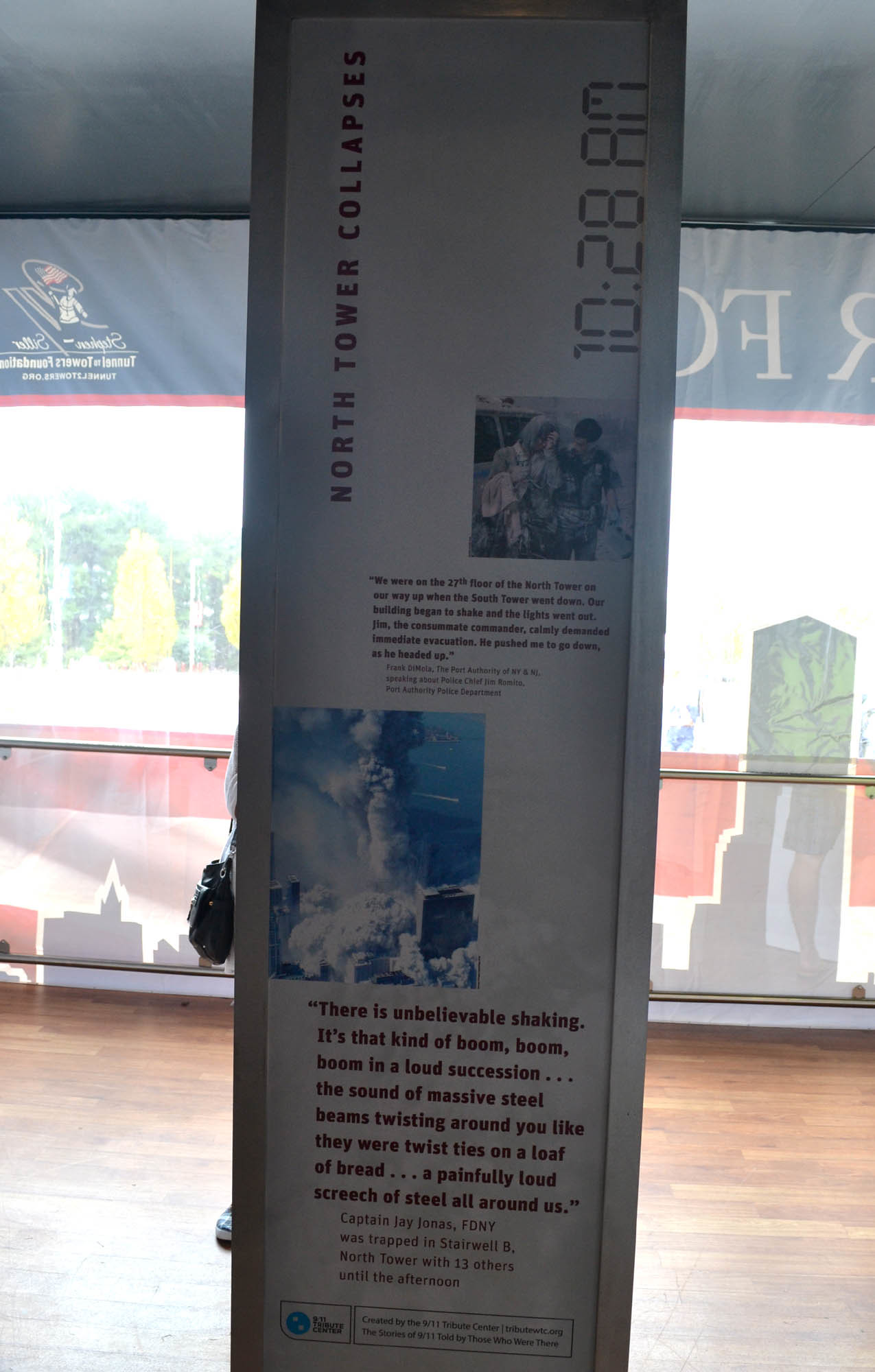The image, reminiscent of a magazine shot, appears to be taken in a museum showcasing a poignant 9/11 exhibit. A central banner
**announces**: "North Tower collapses 10:28." The main sign, encircled by silver horizontal poles with an obscured person in the background, features harrowing quotes. Frank Zamola of the Port Authority of NY and NJ reflects: "We were on the 27th floor of the North Tower going up when the South Tower fell. Our building began to shake; the lights went out. Jim, the consummate commander, immediately demanded evacuation, pushing me to go down as he headed up." Another quote from Captain Jay Jonas, FDNY, captures the chaos: "This is unbelievable. There was an unbelievable shaking, boom boom boom in loud succession, with the sound of massive steel beams twisting like ties on a loaf of bread, and painfully loud screeches of steel all around us. I was trapped in a stairwell of the North Tower with 13 others until the afternoon."